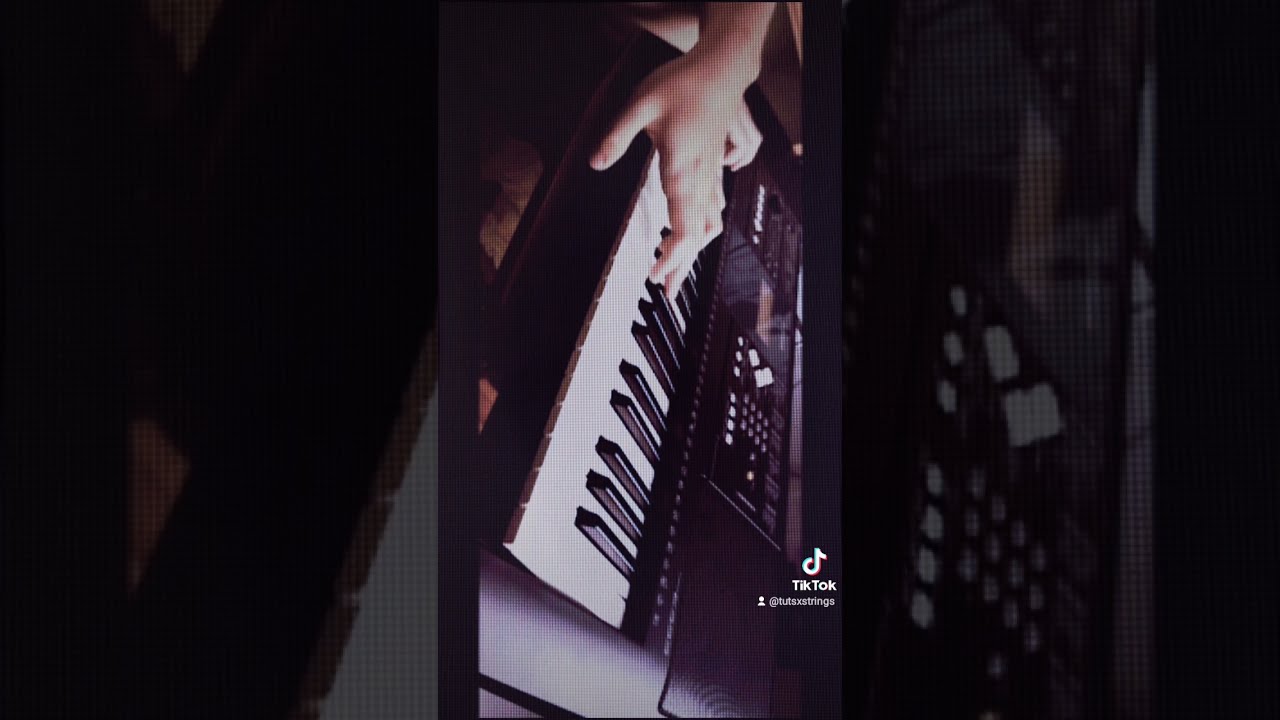The image is a horizontal rectangular screenshot from a video, featuring a close-up of a modern electronic keyboard with white and black keys. The keyboard is being played by two hands, which appear slightly blurry due to movement. The dimly lit setting casts a dark atmosphere over the scene. In the lower right corner of the image, the TikTok logo and address are visible, though the text beneath the logo is unreadable due to its small size. The center of the image, arranged vertically, shows the keyboard at a slightly sideways angle, with visible buttons and an LED screen. To the left and right of this central view, there are blurred close-up sections of the keyboard, one showing part of its edge and the other showing the top area with additional buttons. Built-in speakers are present on both sides of the keyboard, contributing to its sleek, shiny appearance.